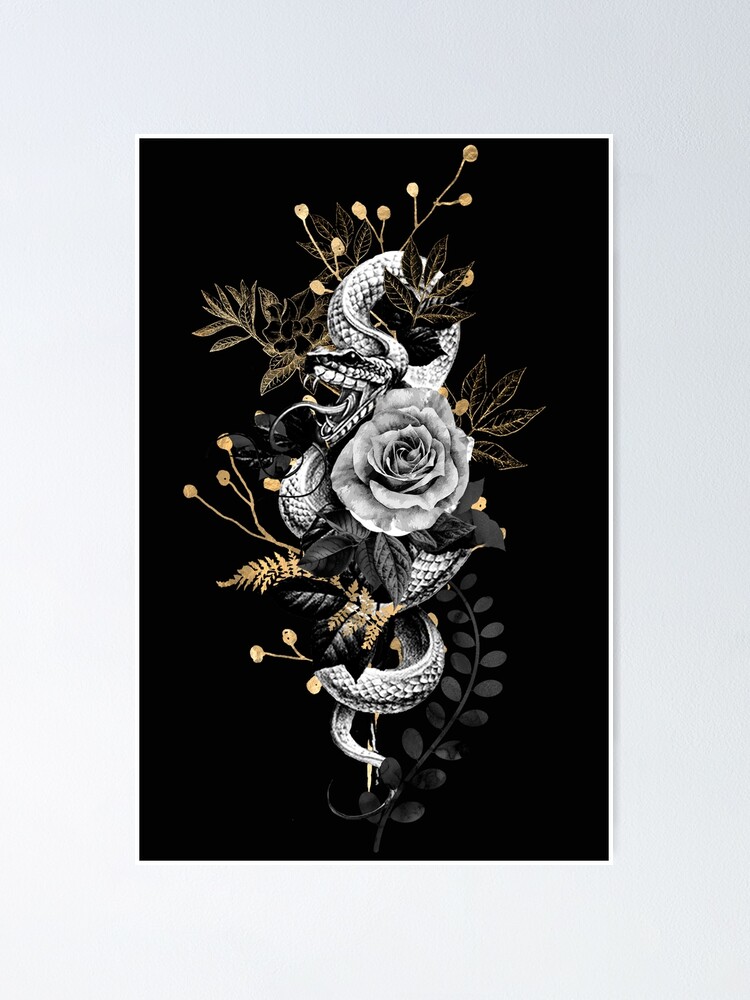The image depicts a vertical piece of artwork with a black background and a thin white border. Dominating the center is a striking black and white sketch of a snake wrapped around a central rose, with the snake’s tail winding around a golden stick and its head positioned at the top, facing left with its mouth open and tongue out, revealing its menacing fangs. This monochromatic serpent contrasts with the surrounding elements, which include additional black and gold roses, green leaves, and small yellow berries and flowers. The intricate details of the snake and floral design create a visually captivating and dramatic composition.